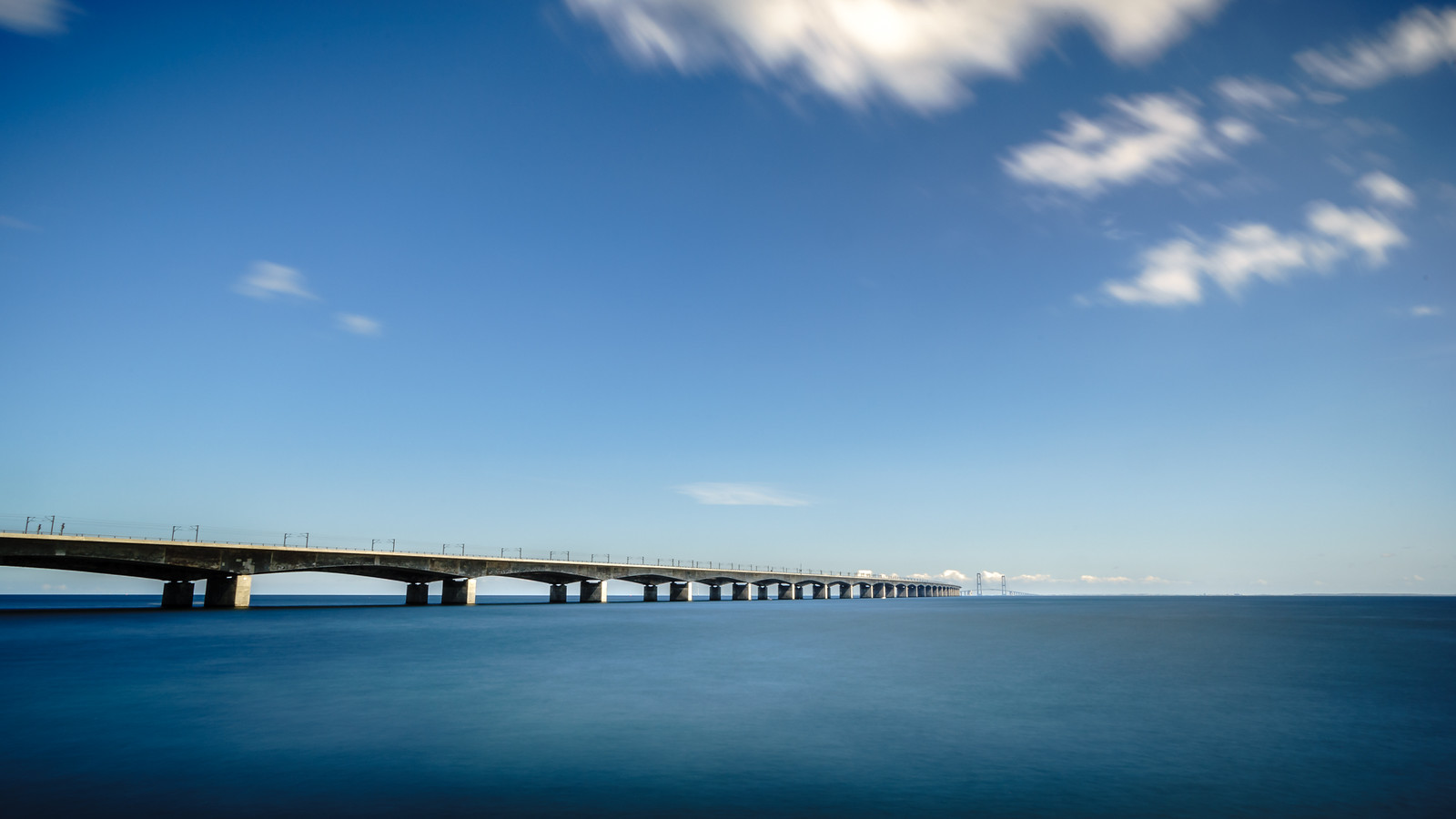This image depicts a long, flat concrete bridge stretching out over the ocean, reminiscent of those found in places like Key West, Florida. The bridge extends into the horizon, so long that its end isn't visible in the photograph. The serene ocean beneath it is a blend of blue and gray hues, while the sky above is clear with white, fluffy clouds scattered across it. Concrete pillars support the structure, ensuring its stability in the water. Both sides of the bridge are edged with fences or support systems to prevent accidents and ensure safety. The image evokes a mix of admiration for the engineering feat and concern for the maintenance and safety of such structures.